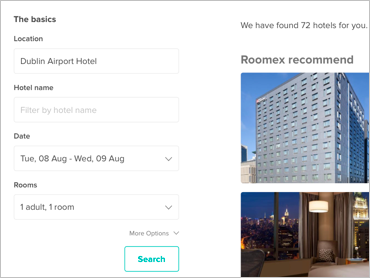The screenshot depicts a web interface for booking a hotel. At the top of the screen, there is a section titled "Basics." Beneath this heading, several information fields are displayed. One field is labeled "Location," with "Dublin Airport Hotel" specified. Another field, labeled "Hotel Name," is currently empty but contains a placeholder text that reads "Filter by hotel name" in a faint gray color.

The date range is presented as "Tuesday, 08 August to Wednesday, 09 August," featuring a drop-down arrow to modify the dates. Additionally, there is a field indicating "1 Adult, 1 Room" which also has a drop-down menu for adjustments. Below this, an option labeled "More Options" is available.

Centered in the interface is a prominent white search button, displaying the word "Search" in a teal color, with the button's border also outlined in teal.

To the right side of the screen, a notice indicates, "We have found 72 hotels for you." Beneath this message, in bold black text, there appears the phrase "Room X Recommend." Directly below, there is an image of a tall, silver-colored hotel building, followed by another image depicting the interior of a room.